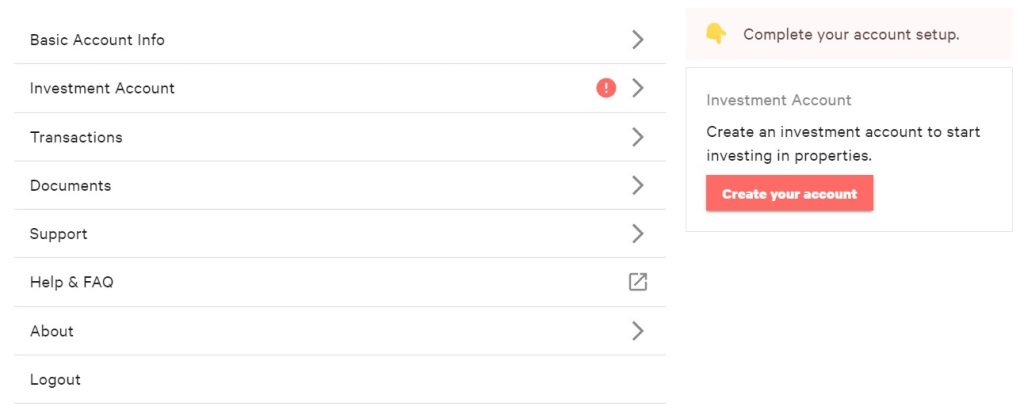The image depicts a webpage interface, primarily featuring typed text in black. The layout is structured in vertical sections, each clearly delineated. At the top of the page is a section titled "Basic Account Info," with a right-pointing arrow at the end of the line for navigation or expansion. Immediately below, the next section is labeled "Investment Account." To the left of this title is a reddish-orange circle containing an exclamation point, indicating an alert or important notice. 

On the right side of the "Investment Account" section, there are two rectangular boxes. The first rectangle has a light pink background and features a gold hand pointing downward, accompanied by the message "Complete your account setup" in black ink. Below this box is another larger reddish-orange horizontal rectangle with white text that reads "Create your account," indicating a call to action for users to proceed with creating their investment account and start investing in properties.